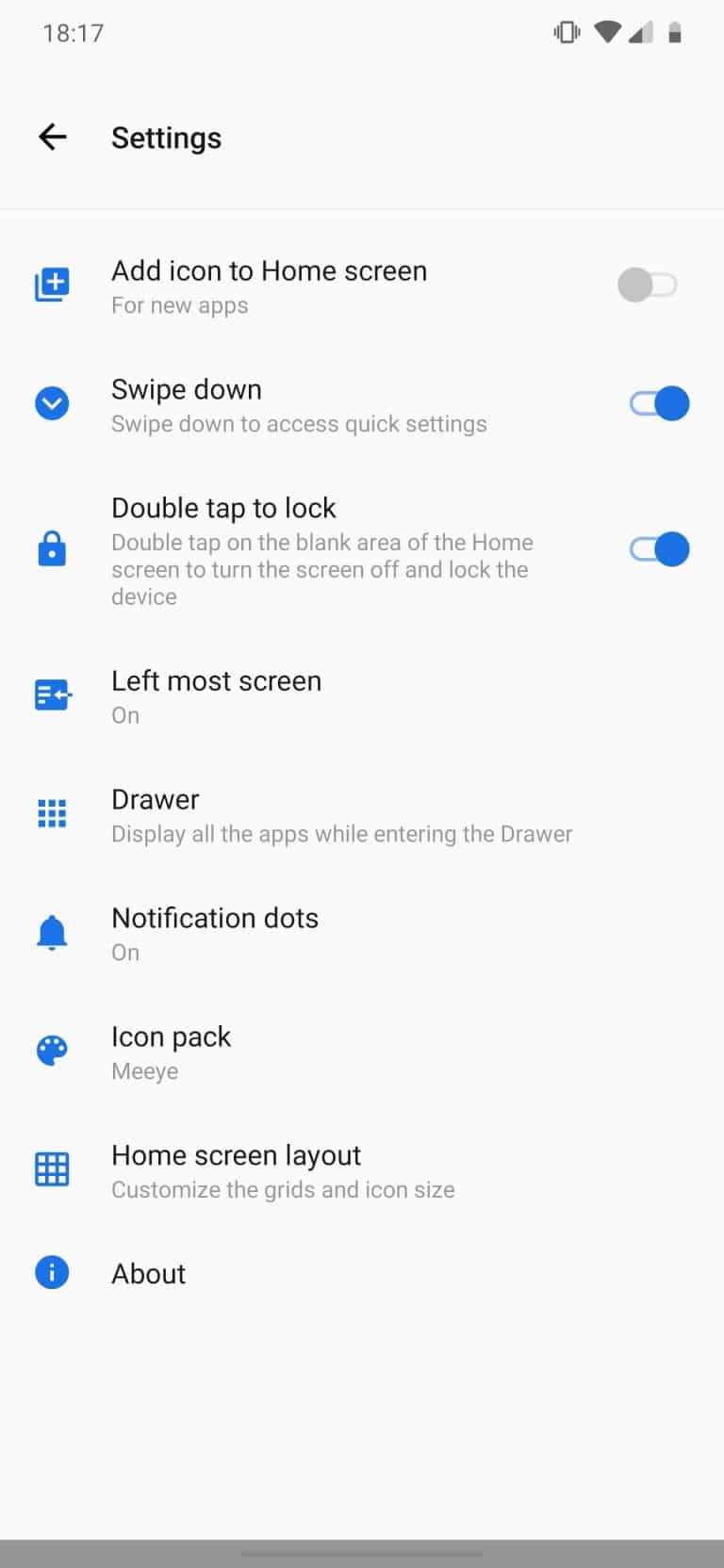The image depicts a screenshot of a smartphone's settings screen against a completely white background. In the upper left-hand corner, the time is displayed as "18:17" in gray text. On the upper right-hand side, there are gray icons indicating the battery level, Wi-Fi signal, and cell signal strength.

Below the time and signal indicators, on the left side, the word "Settings" is prominently displayed in black text, accompanied by a left-pointing arrow, which serves as a back button to navigate to the previous screen.

There are nine different settings options listed vertically, each represented by a blue icon and described in black text. The settings options are:

1. **Add Icon to Home Screen for New Apps**: Represented by a blue square with a white plus sign.
2. **Swipe Down**: Denoted by a blue circle with a white downward arrow.
3. **Double Tap to Lock**: Illustrated by a blue lock icon.
4. **Left Most Screen**: Identified by a blue square with a left-pointing arrow.
5. **Drawer**: Depicted by a grid of nine blue squares.
6. **Notification Dots**: Shown as a blue bell icon.
7. **Icon Pack**: Represented by a blue paint palette icon.
8. **Home Screen Layout**: Iconized by a blue square filled with smaller white squares.
9. **About**: Signified by a blue information icon.

The first three options, "Add Icon to Home Screen for New Apps," "Swipe Down," and "Double Tap to Lock," have toggle switches on the right side. These toggles allow users to enable or disable these features. In the current state, the "Add Icon to Home Screen" toggle is grayed out, indicating that this feature is turned off, while the other two toggles for "Swipe Down" and "Double Tap to Lock" are turned on.